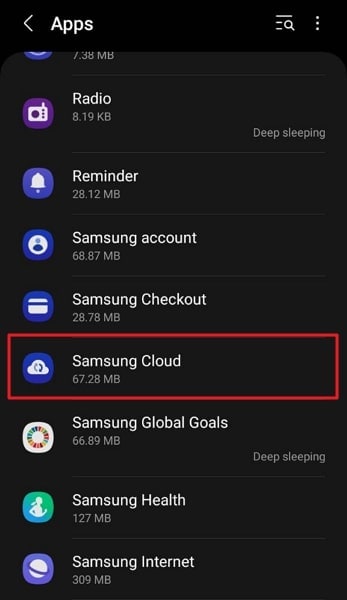The image depicts a menu of apps displayed on a screen with a black background and white text. The first app listed is “Radio,” which is 8.9 KB in size and is represented by an icon of a radio to its left. Next is the “Reminder” app, identified by an icon of a bell. Following that is the “Samsung Account” app, marked by an icon of a person. The “Samsung Checkout” app comes next, denoted by a credit card icon. The highlighted item on the menu is “Samsung Cloud,” which is bordered in red and represented by a cloud icon. Further down the list is “Samsung Global Goals,” accompanied by an unspecified icon. Below it is the “Samsung Health” app, featuring an icon of a runner, and then the “Samsung Internet” app, represented by an internet-icon. The icons for these apps are predominantly displayed within dark blue circles or ovals with the icon itself in white, except for one white circle containing a multicolored icon. There are also green and purple elements within the icon design.